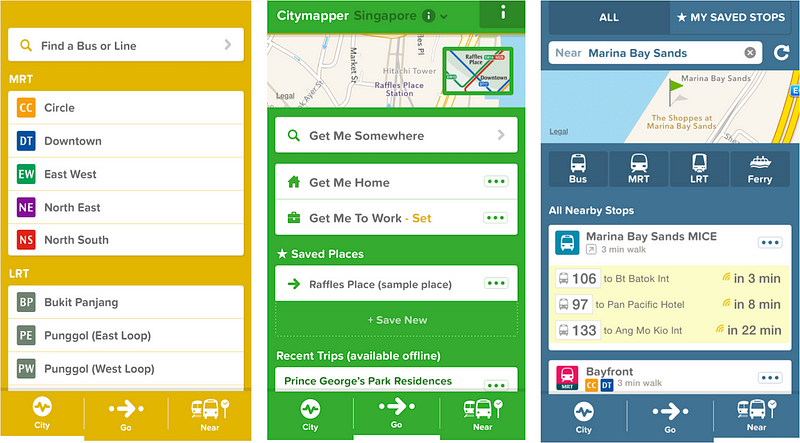This image showcases three mobile phone screens arranged consecutively from left to right, each featuring distinct interfaces and color schemes.

1. **First Screen (Orangey-Yellow Background):**
   - **Top Section:** Features a search bar with the prompt "Find a bus or line."
   - **MRT Section:** Lists several lines including Circle, Downtown, East-West, North-East, and North-South.
   - **LRT Section:** Lists lines such as Bukit, Penang, Punjab (East Loop), and Punjab (West Loop).
   - **Navigation Options at the Bottom:** Includes options named City, Go, and Near.

2. **Second Screen (Green Background):**
   - **Top Section:** Displays a dropdown menu labeled "City map or Singapore."
   - **Map Section:** Below the dropdown is a map view accompanied by a search bar labeled "Get me somewhere" with a right arrow icon.
   - **Quick Access Buttons:** Includes "Get me home" and "Get me to work" for rapid navigation.
   - **Saved Places:** Lists places like "Raffles Place" and "Sample Place," with an option to "Plus Save New."
   - **Recent Trips:** Shows "Prince George's Park Residences" under this section with an indicator that data is available offline.
   - **Bottom Navigation Options:** Features City, Go, and Near.

3. **Third Screen (Blue Background):**
   - **Top Navigation Tabs:** Includes options labeled "All," "Star," "My Saved Stops," and "Near."
   
Each screen is designed to provide comprehensive navigation and transportation information, with specific emphasis on quick access to routes, maps, and saved locations.